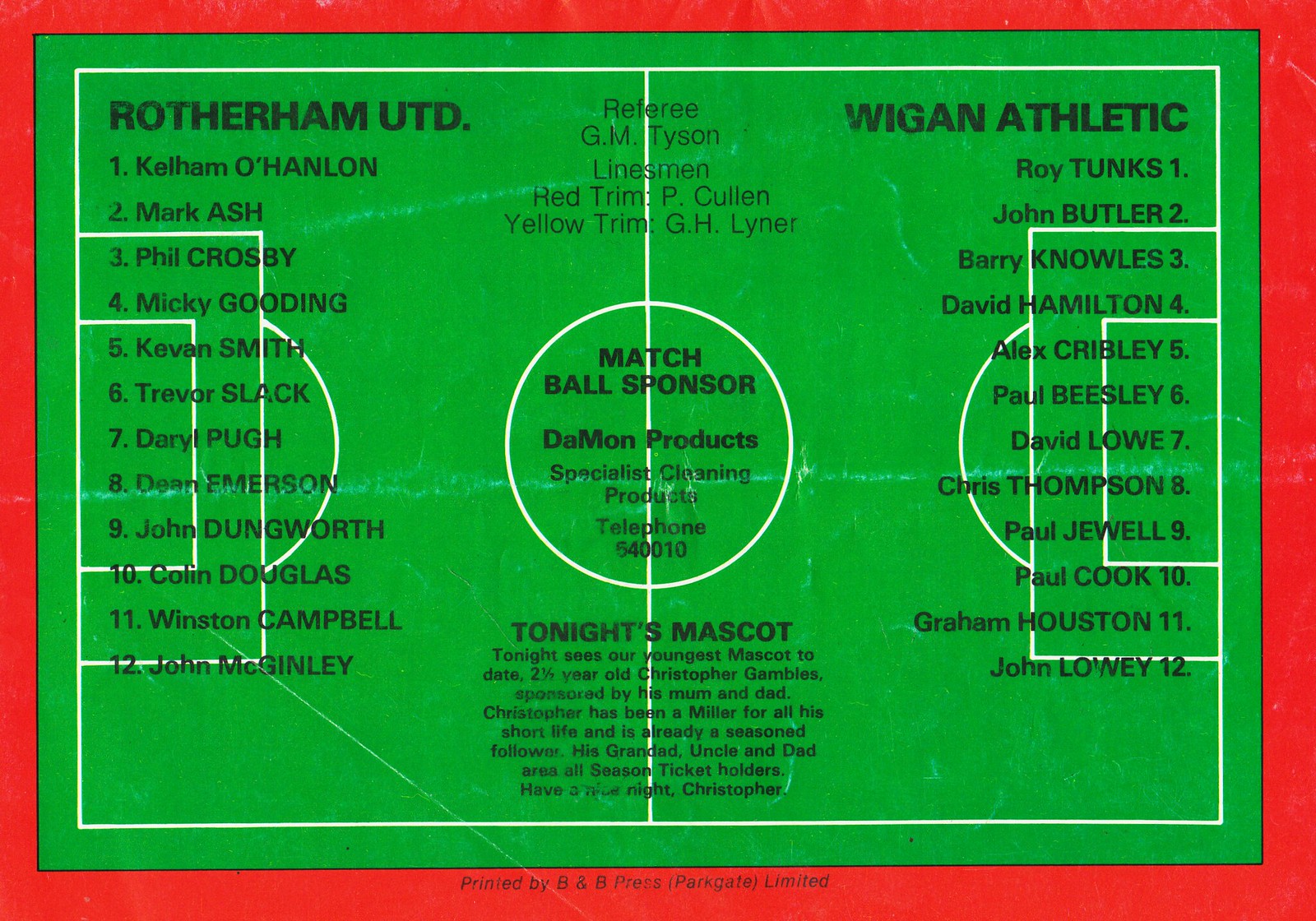This promotional poster for an old soccer match features a computer-generated image of a green soccer field with white lines and a red border. The field diagram is detailed, showing the circles and rectangular goal lines typical of a soccer field but includes no players. The left-hand side lists the players for Rotherham United, including Kelham O'Hanlon and Mickey Gooding, while the right-hand side lists players for Wigan Athletic, such as Roy Tunks and Paul Cook. In the center, a white circle prominently displays the match ball sponsor: Damwon Products, Specialist Cleaning Products, along with a contact telephone number. Above this, the names of the referee and linesman are listed, and below it, there is information about the night’s mascot. The paper itself shows signs of aging, with noticeable fading, creases, and wear marks, indicating it has been folded. The bottom border states "Printed by B&B Press, Parkgate Limited."